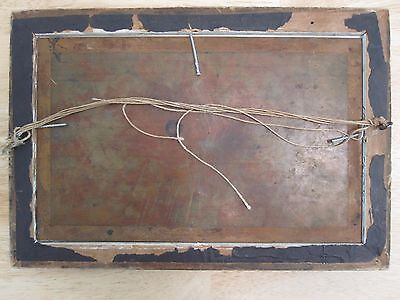The indoor color photograph is a close-up, landscape-style image of the back of a very old, rectangular wooden frame, likely for a picture or painting. The wood of the frame is visibly worn and tattered, with portions of the dark blue paint peeling off to reveal the unfinished light-colored wood beneath. The frame's perimeter is secured with remnants of old tape, indicating past repairs. At the center, a weathered, dirty brown rectangular backing—possibly patinaed metal showing brown and green hues—fills the inner portion of the frame. Two metal mounting clasps are positioned on the left and right sides, connected by a frayed, cream-colored multi-strand twine, which is partially broken and hanging off in pieces. The overall condition suggests the item is an antique, perhaps around a hundred years old.